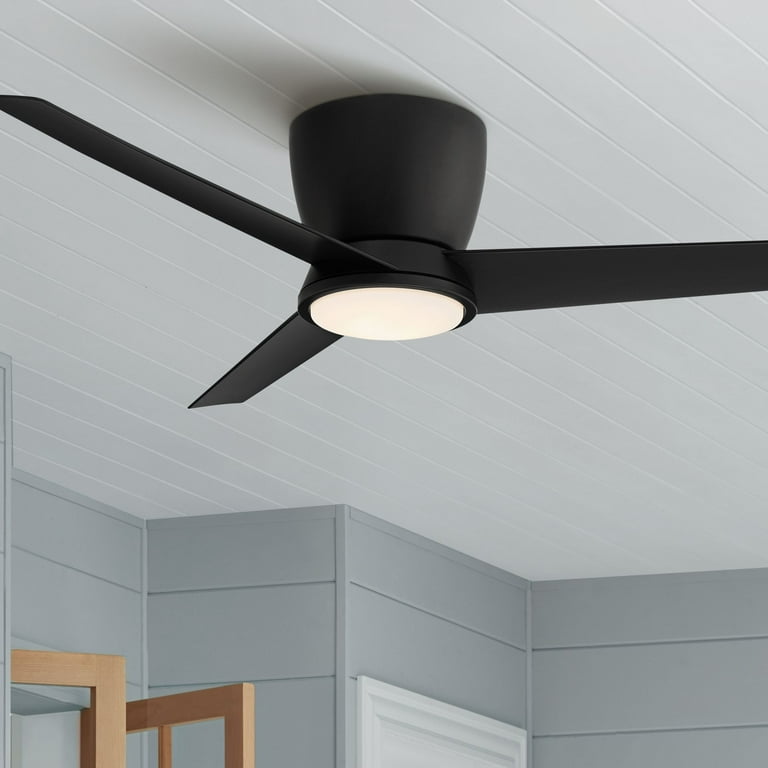The photograph showcases a sleek, modern black ceiling fan with three blades and a centrally located white light fixture, suspended from a thick, vase-like base. The fan is mounted on a white, wooden-paneled ceiling with boards running diagonally from the top left to the middle right of the image. The walls surrounding the fan are painted a grayish-blue color, featuring multiple turns and angles, creating a segmented or divided appearance. In the lower left corner, the image reveals a set of wooden-framed, glass-panel double doors, partially open. Additionally, a white-painted door frame, which seems to lead to a closet, appears in the middle lower section of the photo. The overall room exudes a modern, minimalist aesthetic with its combination of sleek, dark fan elements contrasted against light-colored architectural details.